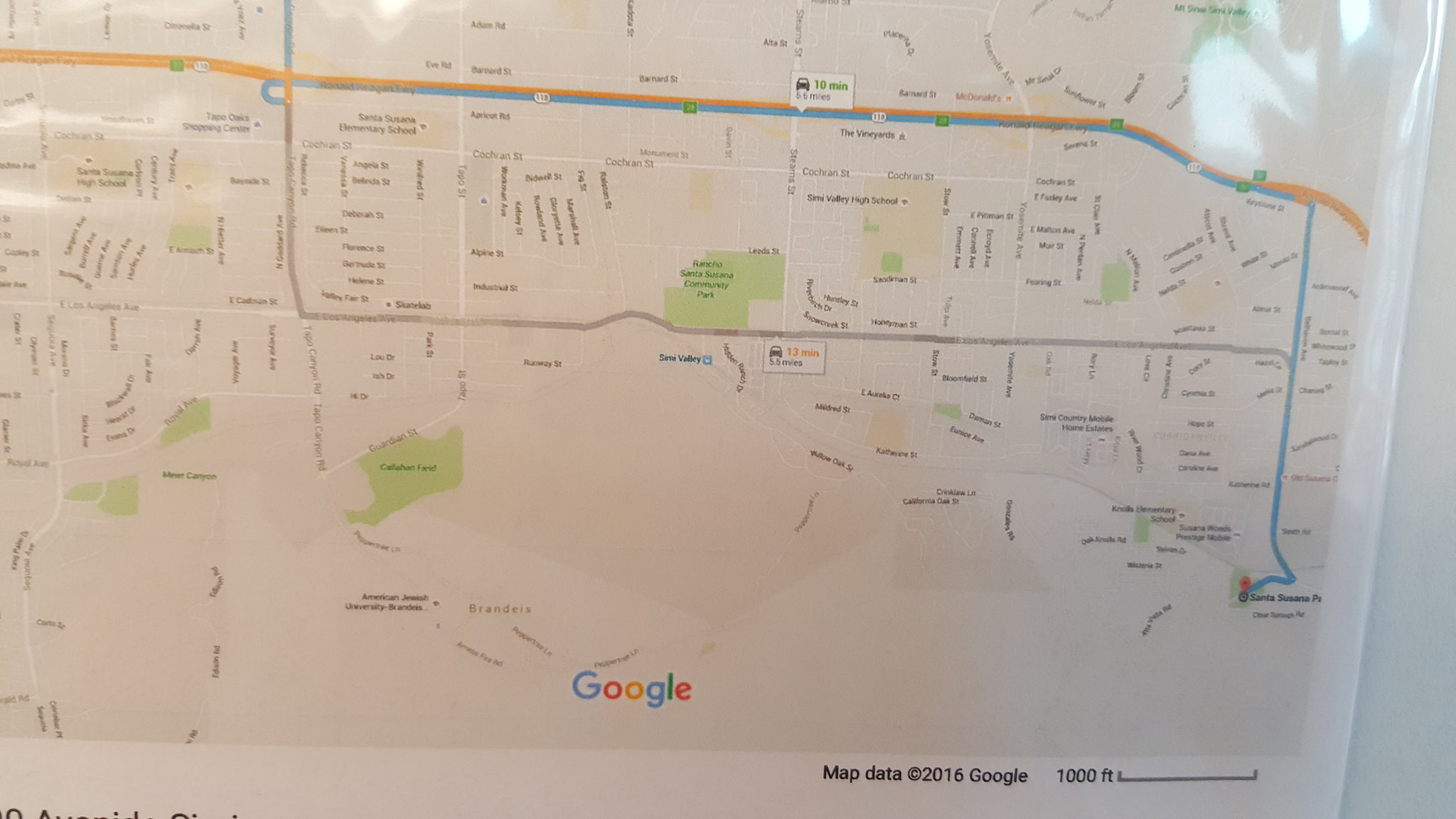This image features a printed Google Map, clearly labeled with copyright information. At the bottom part, black letters read "Map data ©2016 Google" alongside a scale indicator showing "1000 feet." The center-bottom displays the Google logo with its iconic color scheme: yellow "G", red "O", yellow "O", blue "G", green "L", and red "E."

In the top-left corner of the map, an orange-highlighted highway serves as a prominent feature. A blue route traverses this highway, representing a journey estimating travel times as either 18 minutes or 10 minutes. This blue route intersects the highway, proceeds along a main thoroughfare, and eventually terminates in areas marked in red and green.

Adjacent to the yellow-highlighted highway, the blue route is distinct and easily traceable as it moves towards the right side of the map. This specific path guides travelers to their destination, neatly indicated within the indoor setting portrayed on the map.